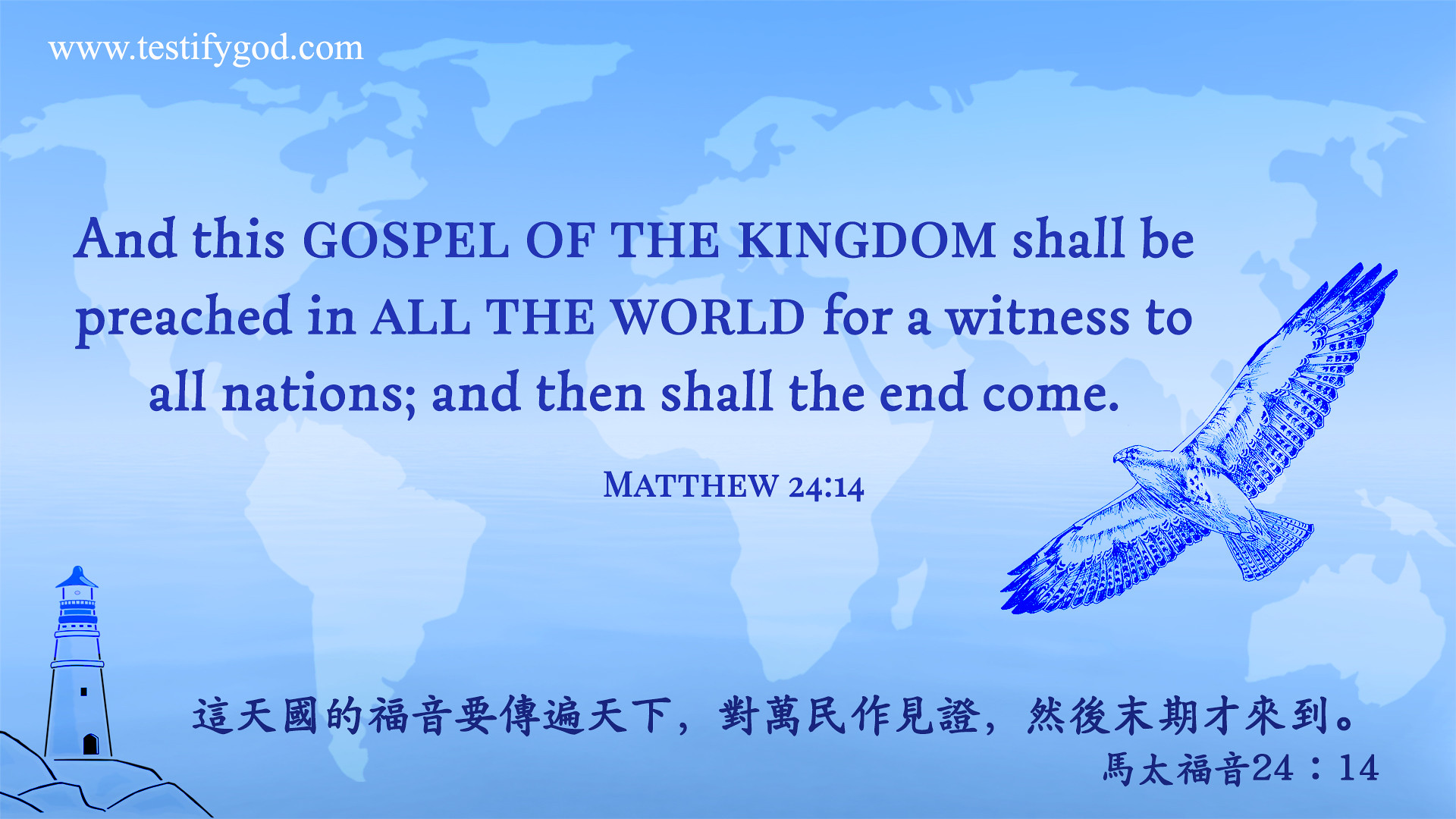The image appears as a rectangular, landscape-oriented design resembling a business card. The background is in various shades of blue, featuring a simplified, less detailed map of the world, with continents depicted in a lighter blue against a darker blue ocean. In the upper left corner, the text "www.testifygod.com" is written in white. Centrally located is a Bible verse in dark blue text: "And this gospel of the kingdom shall be preached in all the world for a witness to all nations, and then shall the end come. Matthew 24:14," with the phrases "Gospel of the Kingdom" and "All the World" in uppercase. To the lower right of the verse, there is an image of an eagle with open wings soaring upwards. In the lower left corner, there is a depiction of a lighthouse situated on rocks. Below this, Asian characters—resembling hieroglyphs—are inscribed.